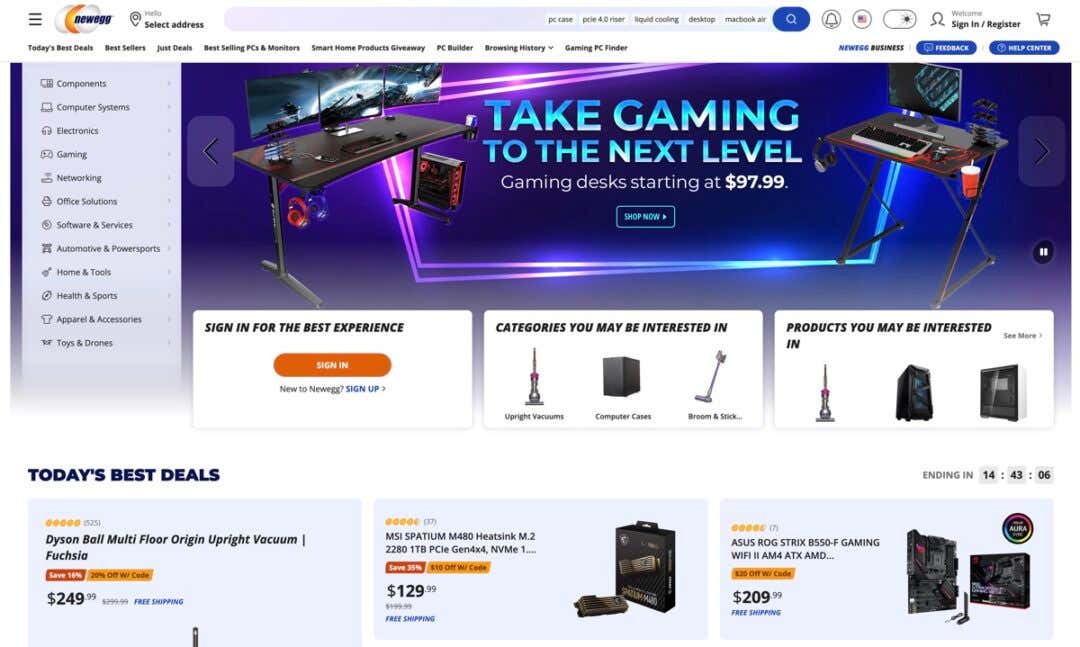**Website Category: Online Retail - Newegg**

At the top of the Newegg website, users will find a navigation bar featuring essential utilities including a search bar, an option to select an address, a notification button, and a USA flag icon. Additionally, there are quick links for signing in or registering an account, as well as accessing the shopping cart. 

On the left-hand side of the webpage is a comprehensive menu listing various categories such as Computer Systems, Components, Electronics, Gaming, Networking, Office Solutions, Software Services, Automotive and PowerPoints, Home and Tools, Health and Sports, Apparel and Accessories, and Toys and Drones.

Prominently displayed is an image with a striking blue background filled with laser lights. The image illustrates a detailed setup featuring a triple monitor arrangement on a primary desk, complemented by an additional computer setup on a smaller desk. Headsets are neatly hanging off the desks, and a drink is placed on one of the desks, adding a touch of personalization.

Beneath this image, the page highlights categories you might be interested in, showcasing items like computer cases and upright vacuum cleaners. Alongside these recommendations, there are several other items displayed with their respective sale prices.